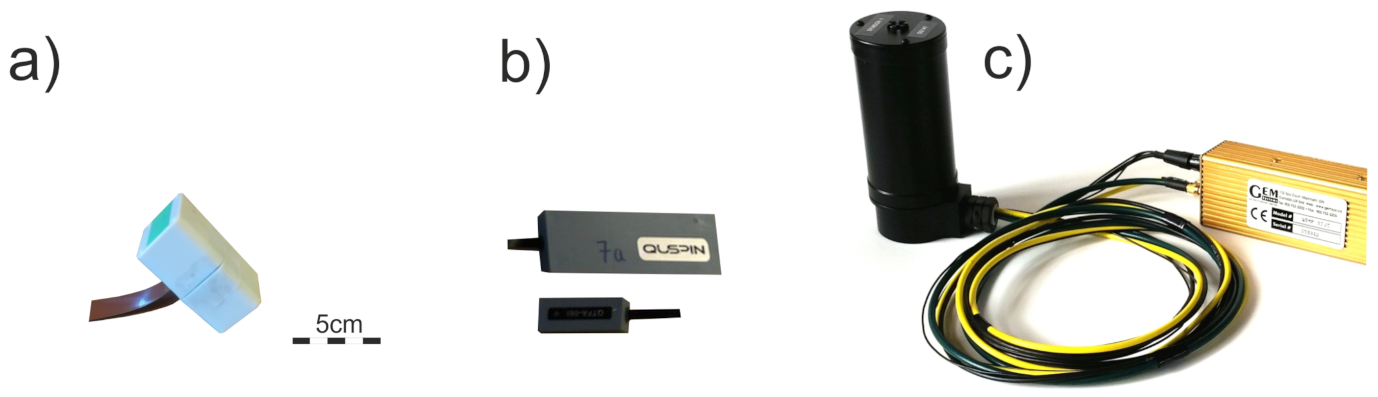This image depicts three electronic components labeled A, B, and C, set against a diagrammatic background. The first object, labeled A, is likely an electrode marked by a notation reading "5 cm" beside it, indicating its size. It consists of a black rectangular piece with a distinctive green section at one end, connected to a dark brown, curved wooden base. A yellow wire connects this part to an orange box. The second object, labeled B, comprises two items: a larger black rectangular panel with a smaller version adjacent to it, appearing to be half or a quarter of its size. Both lack buttons but feature a small antenna extending from them; one of these has handwritten text on a piece of tape affixed to it. The third object, labeled C, resembles a sensor or small camera encased in black, connected via two coiled wires that link to a yellow box with a white label. The wires loop around each other before terminating at the box, suggesting an adapter function. All items are made from a combination of plastic and wires, suggesting their use in an electronic or audio-visual system.